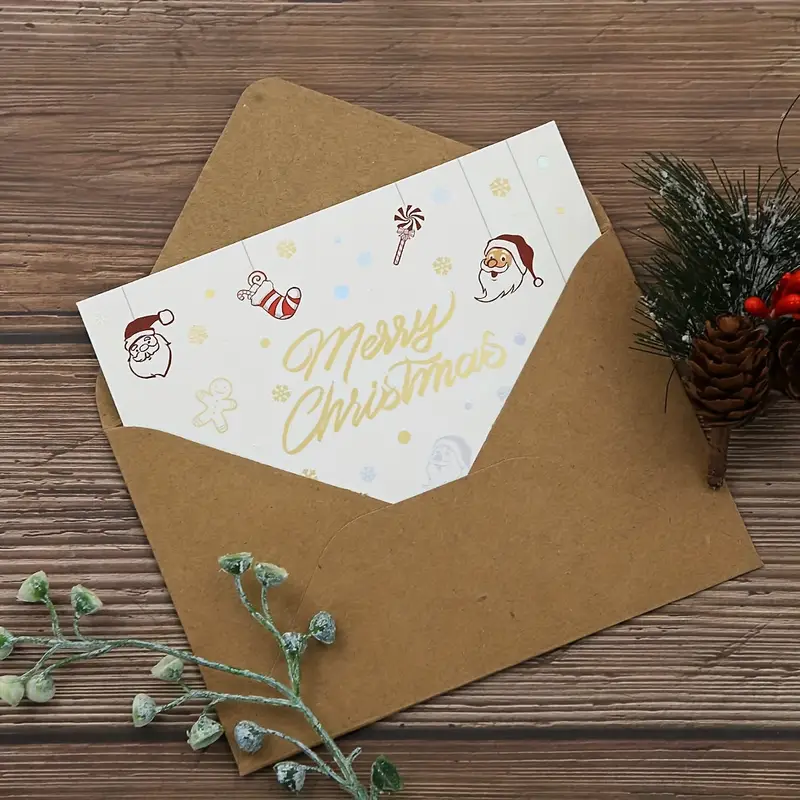A beautifully detailed photograph captures a Christmas card scene set atop a square wooden background. At the heart of the image, a dark tan brown envelope, tilted to the left, reveals a white card partially pulled out. In the center of the card, "Merry Christmas" is inscribed in gold lettering, surrounded by tiny yellow stars and faint snowflakes. The card features festive illustrations: a Santa head, a stocking, a windmill, and another Santa head, all attached to strings from the top, while a faint Santa head can be discerned near the bottom of the envelope. Over on the lower left side, sprigs of a green wintery plant, adorned with green flowers, rest gracefully. On the mid-right side, a pine cone embellished with pine needles and red berries adds a touch of natural charm to the seasonal tableau. This intricate arrangement evokes a warm and festive holiday spirit, perfectly captured in a single frame.